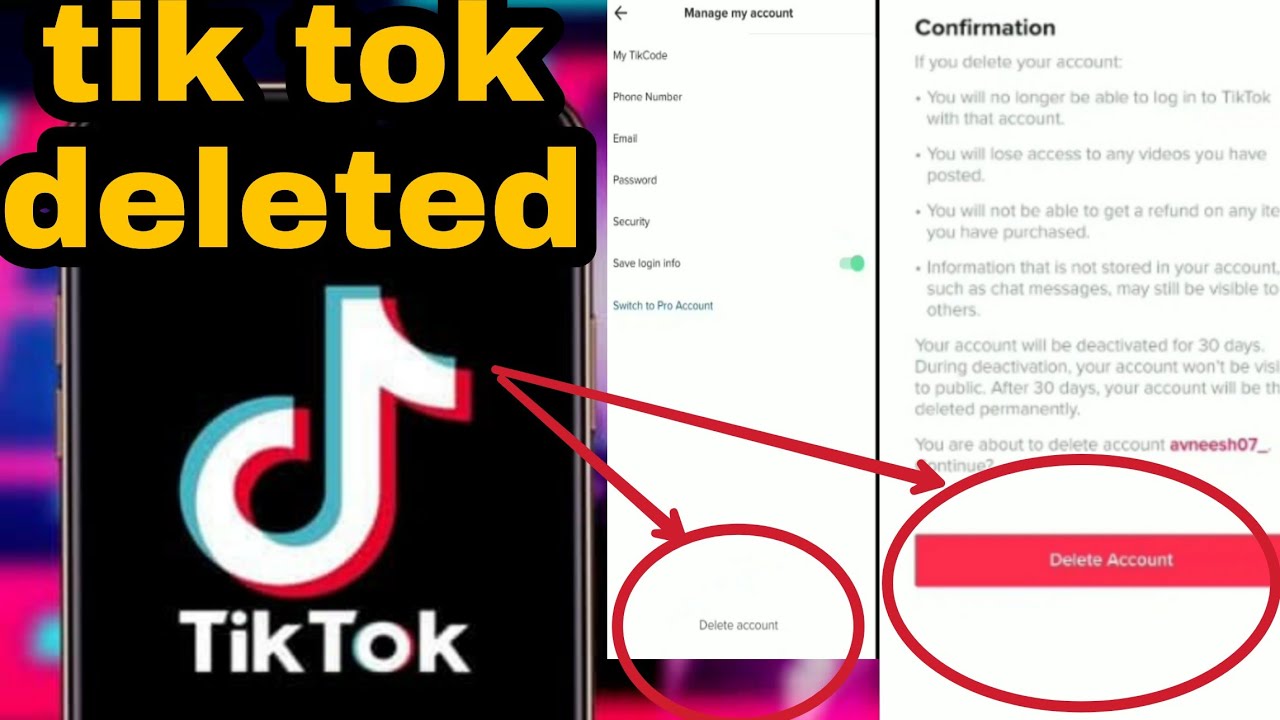The composite image consists of three adjacent screenshots. The first image features the recognizable TikTok logo against a black background. Bold yellow text with a black drop shadow hovers above the logo, stating "TikTok Deleted." From this image, two red arrows extend to the right, directing attention to the middle screenshot.

The second image displays a white background with black text reading "Manage My Account." This section encapsulates various account settings, including options to view your TikTok code, update your phone number, email, and password, and adjust security settings. It also has options for login information and switching to a pro account. The focus of this screenshot, however, is a circled "Delete Account" button, highlighted by an arrow from the left image.

The third image, on the far right, has a white background with black text that serves as a confirmation prompt. This text explains the consequences of deleting a TikTok account: loss of access to the account and videos, inability to obtain refunds on purchased items, potential visibility of chat messages to others, and a 30-day deactivation period before permanent deletion. Highlighting the imminent action, the username "AVNEESH07" is presented in pink. Below this, a large red button labeled "Delete Account" is prominently circled, urging final confirmation of the deletion.